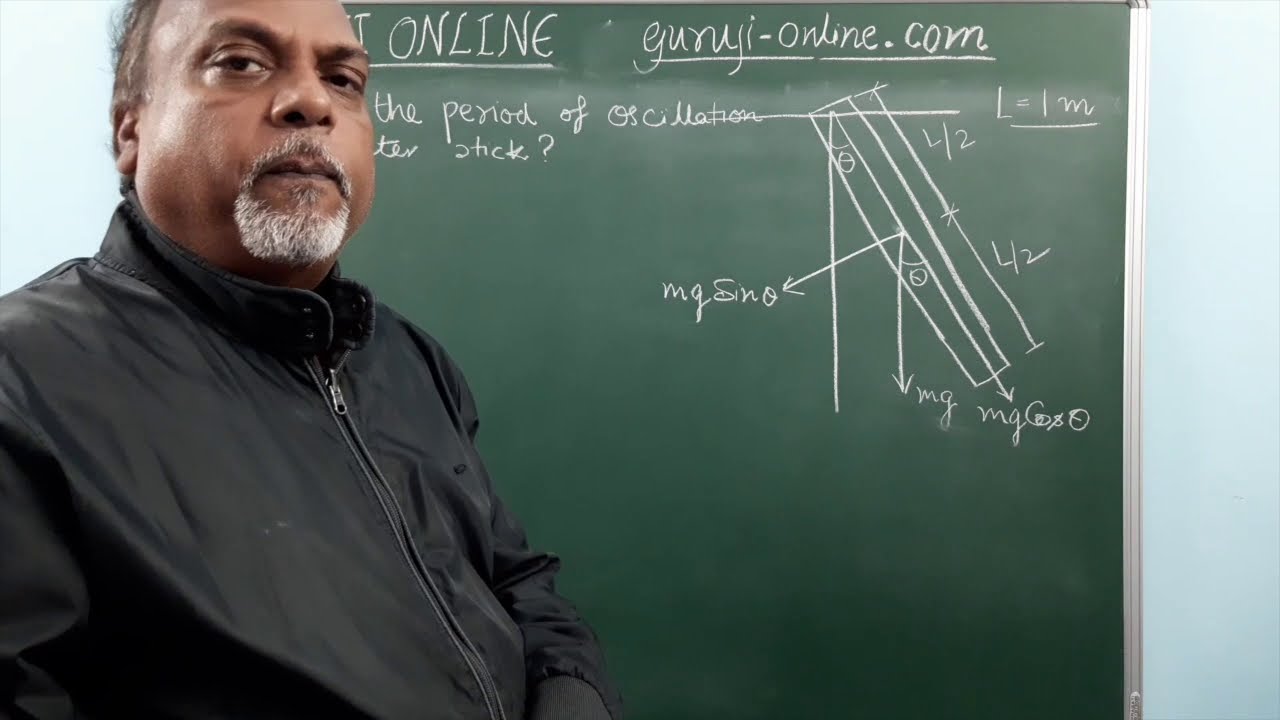The image depicts a man, reminiscent of Neil deGrasse Tyson with a slightly frustrated expression, standing in front of a green, metal-framed chalkboard. He has dark skin, brown eyes, a white mustache and goatee, and what appears to be thinning hair, though the top of his head is out of the frame. The man is wearing a long-sleeve, black zip-up jacket without a hood. The chalkboard has various writings in white chalk, including the partially obscured phrases "gun-e-online.com" and "period of oscillation," as well as the word "online" clearly visible. There are also geometric figures and possibly measurement-related diagrams, such as a tilted ruler. The background wall appears light blue, and the image captures him from the waist up, suggesting a university professor setting.